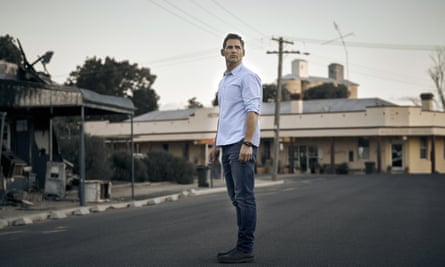In the center of the photograph stands a man, likely in his 30s or 40s, with brown hair. He's clad in a white, long-sleeved button-up collared shirt, which is rolled up to reveal most of his lower arms, and accessorized with a black watch. His outfit is completed with black jeans and black boots. He stands on a dark, almost black asphalt road, gazing off into the distance. 

The background reveals a richly detailed urban scene. To the left of the man is a canopied entrance leading to a dilapidated building with a metal roof supported by thin poles. The sidewalk in front of this building is cluttered with what appears to be damaged or discarded items, possibly burned or destroyed. Adjacent to this scene is a cream-colored building with a metal roof, seemingly in better condition. 

Further in the distance, a much taller building with two prominent higher sections looms over the scene. Power lines stretch to the left, right, and above the man's head, connected to a wooden power pole in the vicinity. The muted, almost desaturated tones of the photograph, paired with a grey sky, imbue the image with a somewhat somber atmosphere.